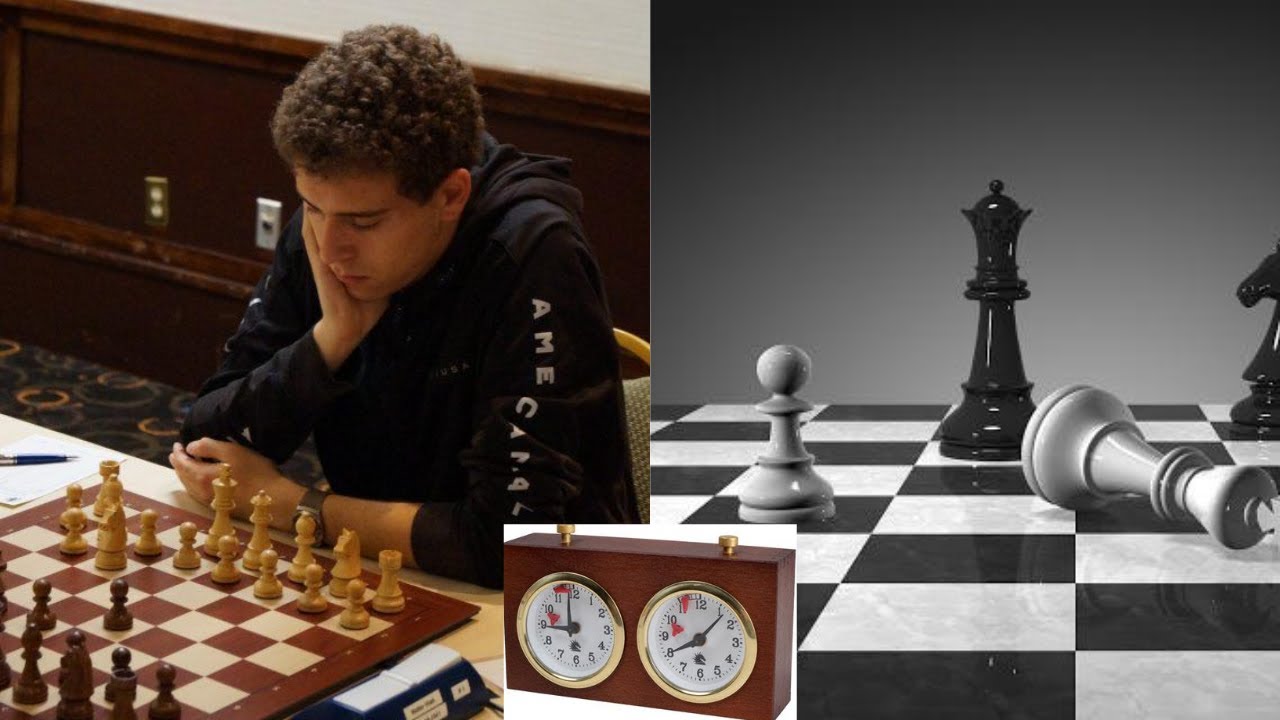The combined image showcases a moment from a chess tournament through two primary pictures along with a smaller supplemental photo. The left image, in color, features a young man with short curly hair, dressed in a black hoodie with rolled-up sleeves. He's deeply engrossed in the game, leaning on the table with his head resting on his hand, intently studying the chessboard before him. His side, represented by the white pieces, has made some moves, but the opposing black pieces appear to be advancing more aggressively. In contrast, the right image is a grayscale close-up of a chessboard, where a toppled white queen lies before a standing king and pawn, suggesting a moment of defeat. Both main images are unified by a traditional chess clock situated at the bottom center, emphasizing the critical time element in competitive chess.